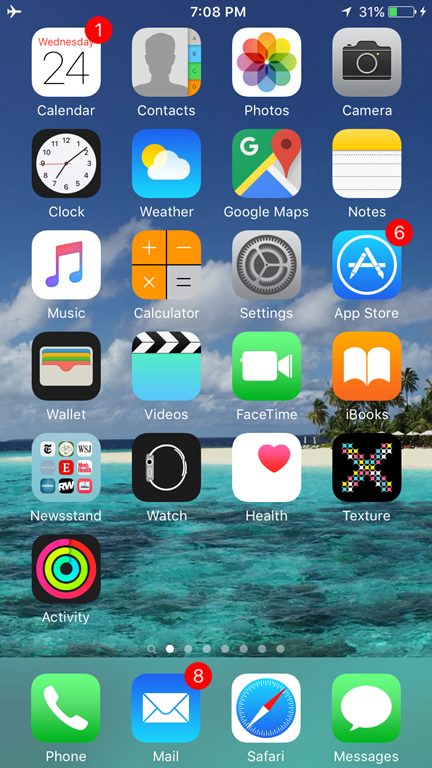The image features a mobile phone screen with a blue background. At the top left, the phone is in airplane mode. The current time, displayed in white, is 7:08 PM, situated in the middle of the screen. A battery icon on the right indicates a 31% charge, accompanied by a lightning bolt symbol suggesting charging. The date, Wednesday 24th, is highlighted in red.

Below the status bar, the screen displays several app icons arranged in rows. From left to right, top to bottom, the apps are as follows:

1. **Messages App**: Indicated by a red circle with one unread message.
2. **Calendar**: Marked with the date "24".
3. **Contacts**: Represented by a gray silhouette of a person on a white background.
4. **Photos**: Featuring the NBC peacock logo, resembling a colorful flower.
5. **Camera**: Depicted by a black camera icon on a gray background.
6. **Clock**: A standard clock icon.
7. **Weather**: Blue background with yellow and white cloud imagery.
8. **Google Maps**: Icon with a 'G'.
9. **Notes**: Yellow top with white lined paper at the bottom.
10. **Music**: Noted by a red and blue music note.
11. **Calculator**: Orange and gray icon.
12. **Settings**: Gray gear circle icon.
13. **App Store**: Blue icon with a white circle and 'A'. A red circle indicates six notifications.
14. **Wallet**: Represented by a wallet icon.
15. **Videos**: An action clip, black and white, with a light blue background.
16. **FaceTime**: White camera on a green background.
17. **iBooks**: Orange background with a white book icon.
18. **Newsstand**: Featuring an assortment of newspapers on a gray background.
19. **Watch**: Gray watch on a black background.
20. **Health**: White background with a red heart on the right.
21. **Texture**: Black background with a large white 'X'.
22. **Activity**: Black background with concentric circles colored red, green, and blue, with a black center.

At the bottom of the screen are four frequently used apps:
- **Phone**: Green icon with a white phone.
- **Mail**: White envelope on a blue background, showing 8 unread messages in a red circle.
- **Safari**: Blue circle with a red and white compass on a white background.
- **Messages**: Green background with a white speech balloon.

The background image of the home screen shows a green water scene with a white sandy beach, a few green trees to the right, and blue sky with gray clouds. The base of the screen has a textured green area.